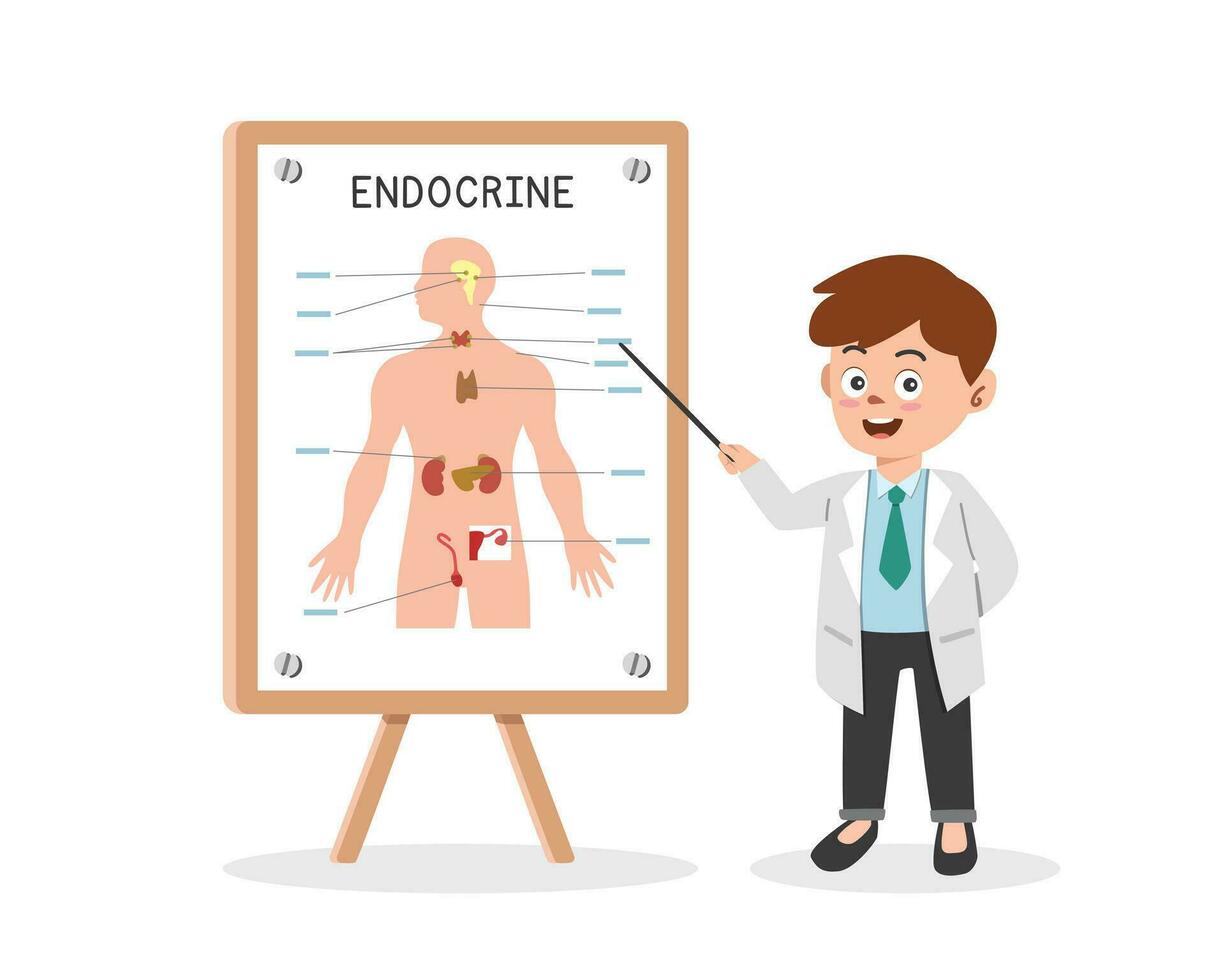The image showcases a computer-generated graphic of a male physician. He is dressed in black jeans and black shoes resembling loafers. He also wears a blue dress shirt paired with a greenish-teal tie, topped with a white lab coat. The avatar has brown hair and is depicted holding a wand-like instrument in his right hand, which he uses to point at a wooden board. The board features a white poster with the word "Endocrine" written on it and displays a human figure with various anatomical parts labeled.